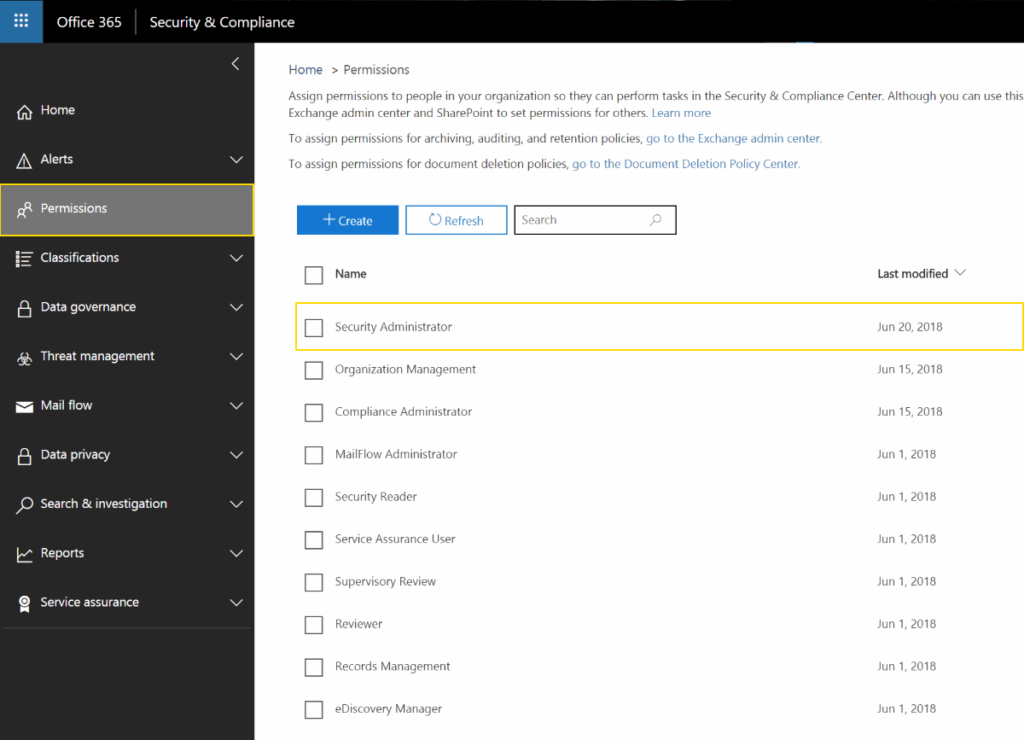The image depicts the user interface of Office 365, specifically focusing on the Permissions section within the Security and Compliance Center. On the left, there is a black pane with white text containing various navigation options: Home, Alerts, Permissions, Classifications, Data Governance, Threat Management, Mail Flow, Data Privacy, Search and Investigation, Reports, and Service Assurance. 

The user has selected the "Permissions" option, which brings up detailed information on the right side. This section is dedicated to assigning permissions to individuals within an organization, enabling them to perform specific tasks related to security and compliance. The description highlights possible actions, such as using the Exchange Admin Center and SharePoint for setting permissions. The interface suggests that Office 365 integrates various tools, including Exchange, to facilitate these tasks.

Additionally, a list of roles is visible, including Security Administrator, Organization Management, and Compliance Administrator, indicating that these roles can be modified or assigned to different users. The environment appears to be designed for a network of business professionals, aimed at managing user privileges and administrative roles efficiently.